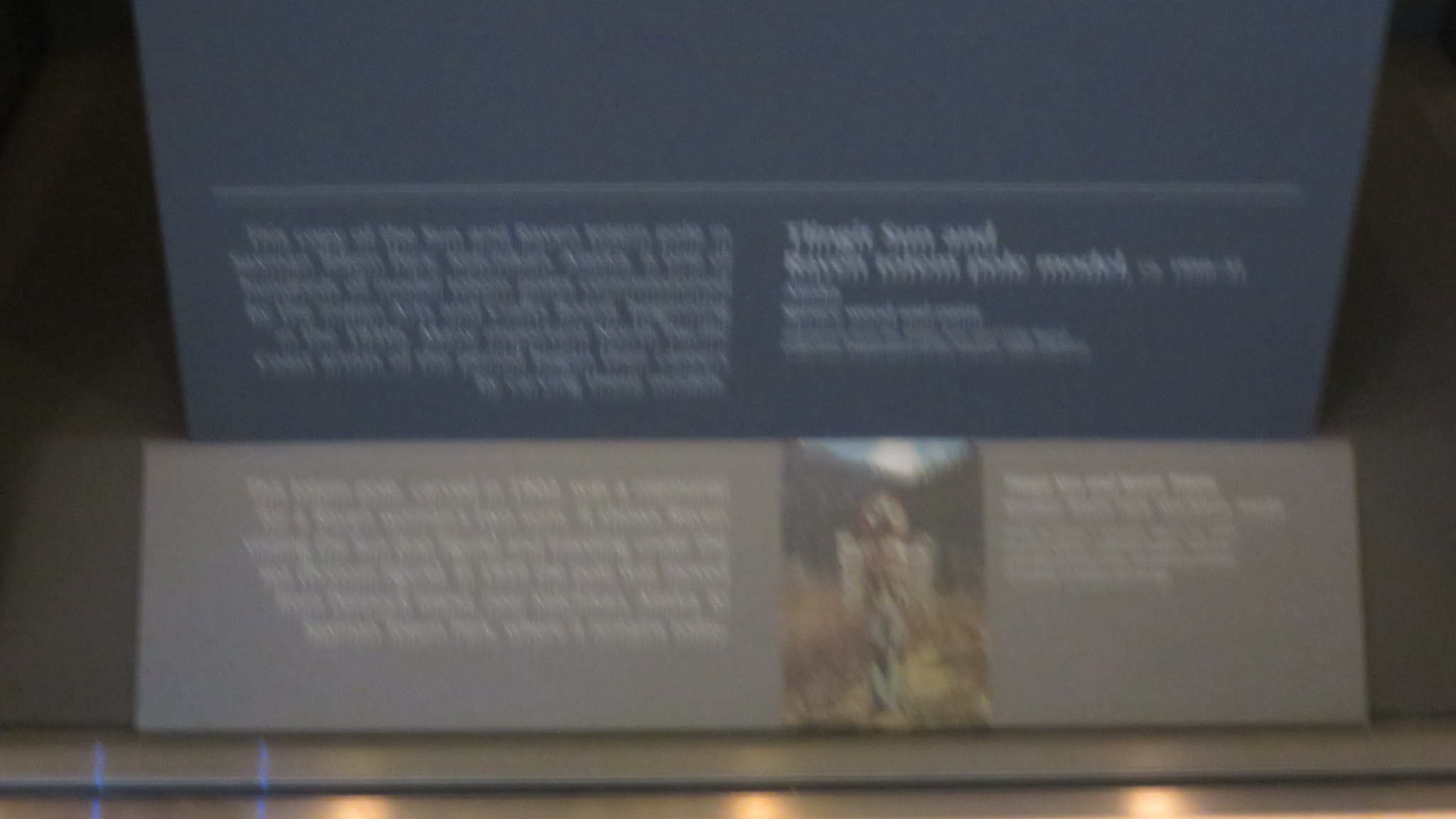In the center of the image, there is a figure standing against a backdrop. At the very bottom of the image, there is a gray panel featuring an information section. On the left side of this panel, there is a paragraph of text, detailing some information. Just above this panel, an image appears to include an individual standing. To the right of this central figure, more text is visible, followed by another gray square. Moving upwards in the scene, the top portion of the image is marked by a blue rectangle intersected by a white line with a point at the cross. The left side of the image contains another paragraph, while the right side has text that includes words like "sun" and another part that is difficult to read. The text on the right side through a paragraph likely contains a description, title, or byline. Both the far left and right edges of the image are dark. The bottom of the image showcases light sources reflecting off metallic surfaces. The composition hints at an organized layout featuring informational text and visual elements.